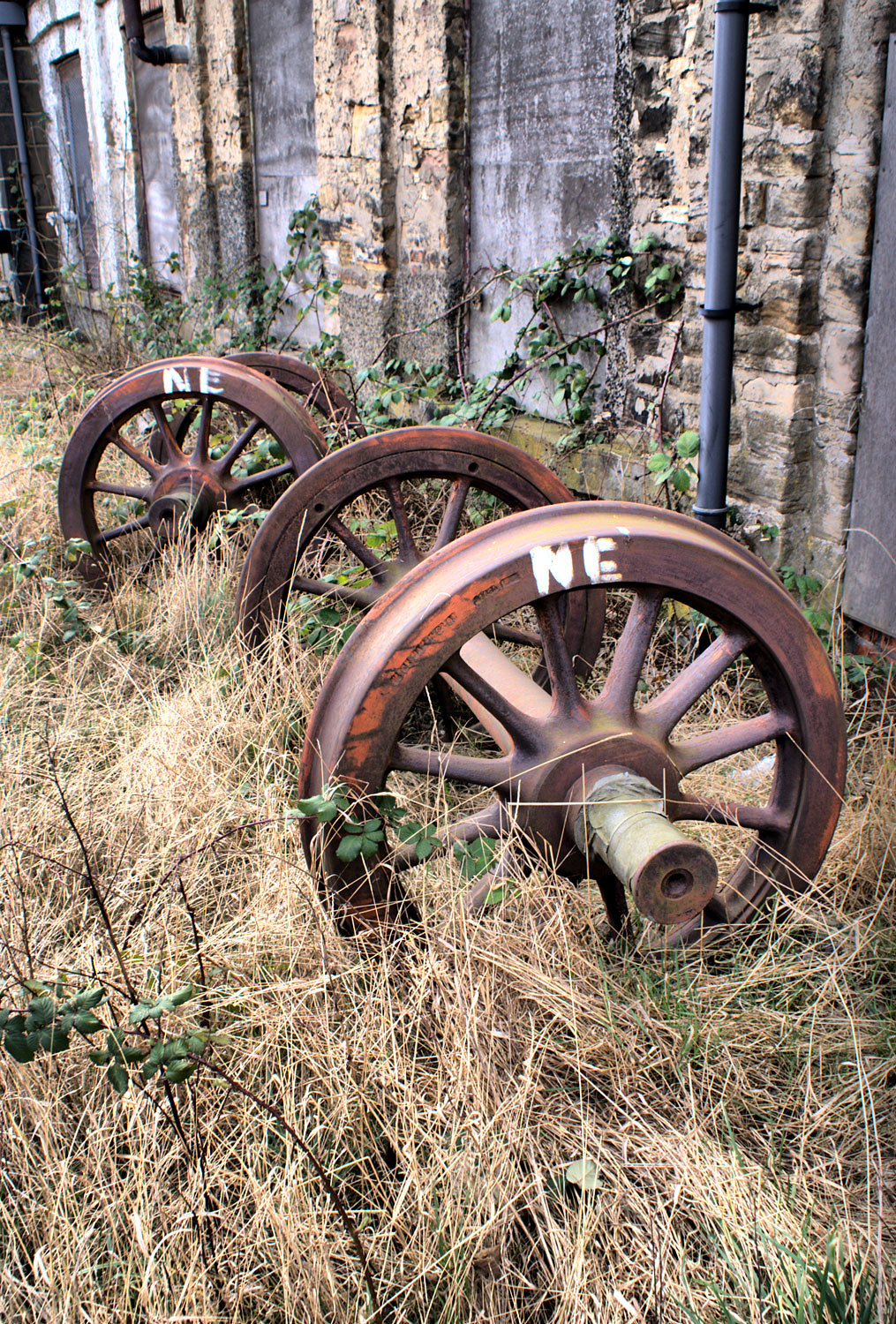This outdoor scene depicts an old, weathered stone wall made of gray and beige bricks, interspersed with black patches and a chipping surface suggesting age and neglect. The backdrop includes a metal black pipe protruding from the wall and a vine creeping up its face. At the base of the wall, long, dry, brown and wheat-colored grass mingles with green twigs. Dominating the center of the image are at least two pairs of rusty, orangey-red metal wagon wheels from a bygone era, potentially over a hundred years old. Some of these wheels feature white-painted "N.E." letters. The wheels have spokes and protruding attachments, indicating they were likely used in conjunction with old buggies or wagons. The scene captures a sense of abandonment and historical decay.